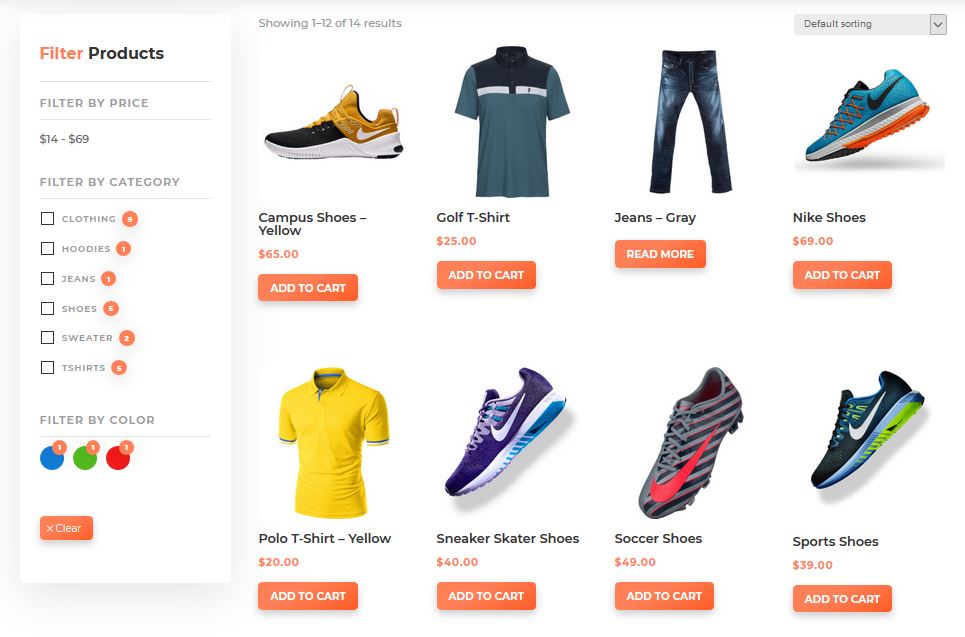**Website Product Page Description:**

This webpage features a detailed product filtering and display system for an apparel and footwear e-commerce store. On the left-hand side, the filtering options allow users to narrow down their search by various criteria:

- **Filter by Price:** Users can specify a price range from $14 to $69.
- **Filter by Category:** Categories include clothing, hoodies, jeans, shoes, sweaters, and t-shirts.
- **Filter by Color:** Available color options are blue, green, and red.
- **Clear Filters Button:** At the bottom of the filter sidebar, users can reset all filters.

On the right-hand side of the page, products are displayed. The page currently shows 1 to 12 out of a total of 14 results. The listed products include:

1. **Campus Shoes Yellow:** Black and yellow sneakers.
2. **Golf T-shirt:** Dark blue with a white stripe and teal accents.
3. **Jeans Gray:** Clearly stonewashed jeans in varying colors, with no specified price.
4. **Nike Shoes:** Priced at $69.
5. **Polo T-shirt Yellow:** $20. This yellow short-sleeve shirt features blue lines around the cuffs of the arms.
6. **Sneaker Skater Shoes:** Priced at $40.
7. **Soccer Shoes:** Priced at $49.
8. **Sports Shoes:** Priced at $39.

The product descriptions provide an informative overview, helping users make informed purchasing decisions.